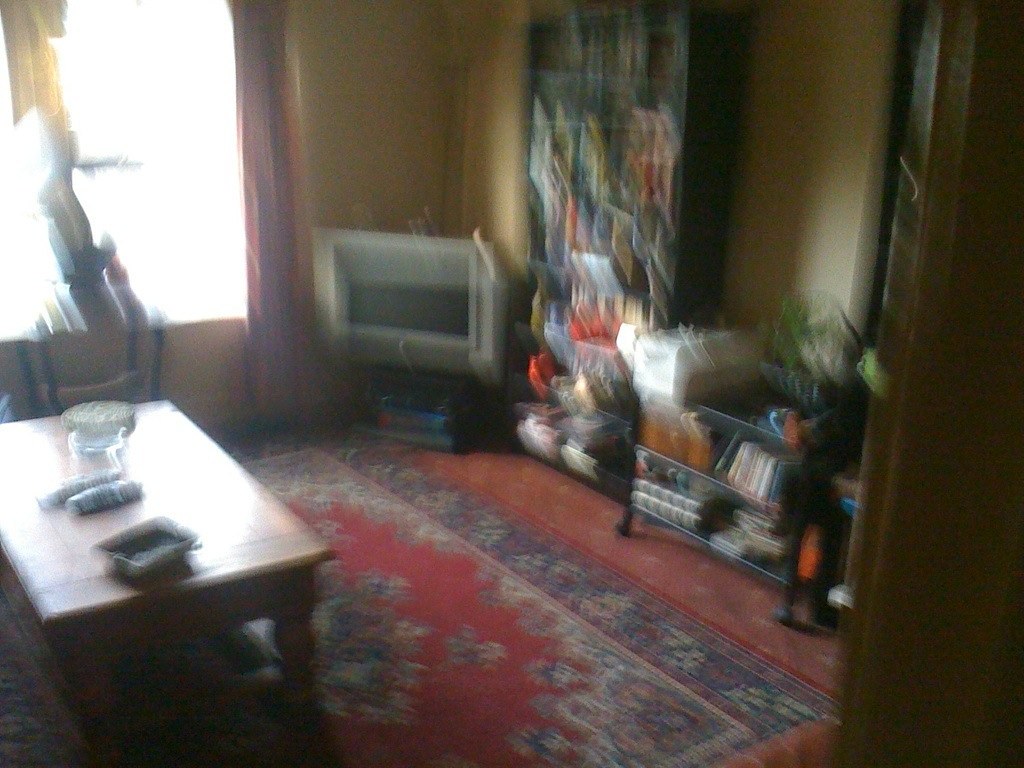In this blurred image of a retro-themed living room, the left side features a wooden coffee table reminiscent of 1970s-80s design. Atop the table rests a small gray dish and a clear mason jar-like container. Adjacent to the coffee table, an end table stands against a wall with a brightly illuminated window, indicating daylight. The floor is adorned with a traditional Oriental-style rug, predominantly red with floral motifs in various colors, especially blue. Along the far wall in the corner is an old 32-inch CRT television with a gray border. Next to the TV is a bookshelf and a smaller bookshelf with a plant on top, both filled with an assortment of books.